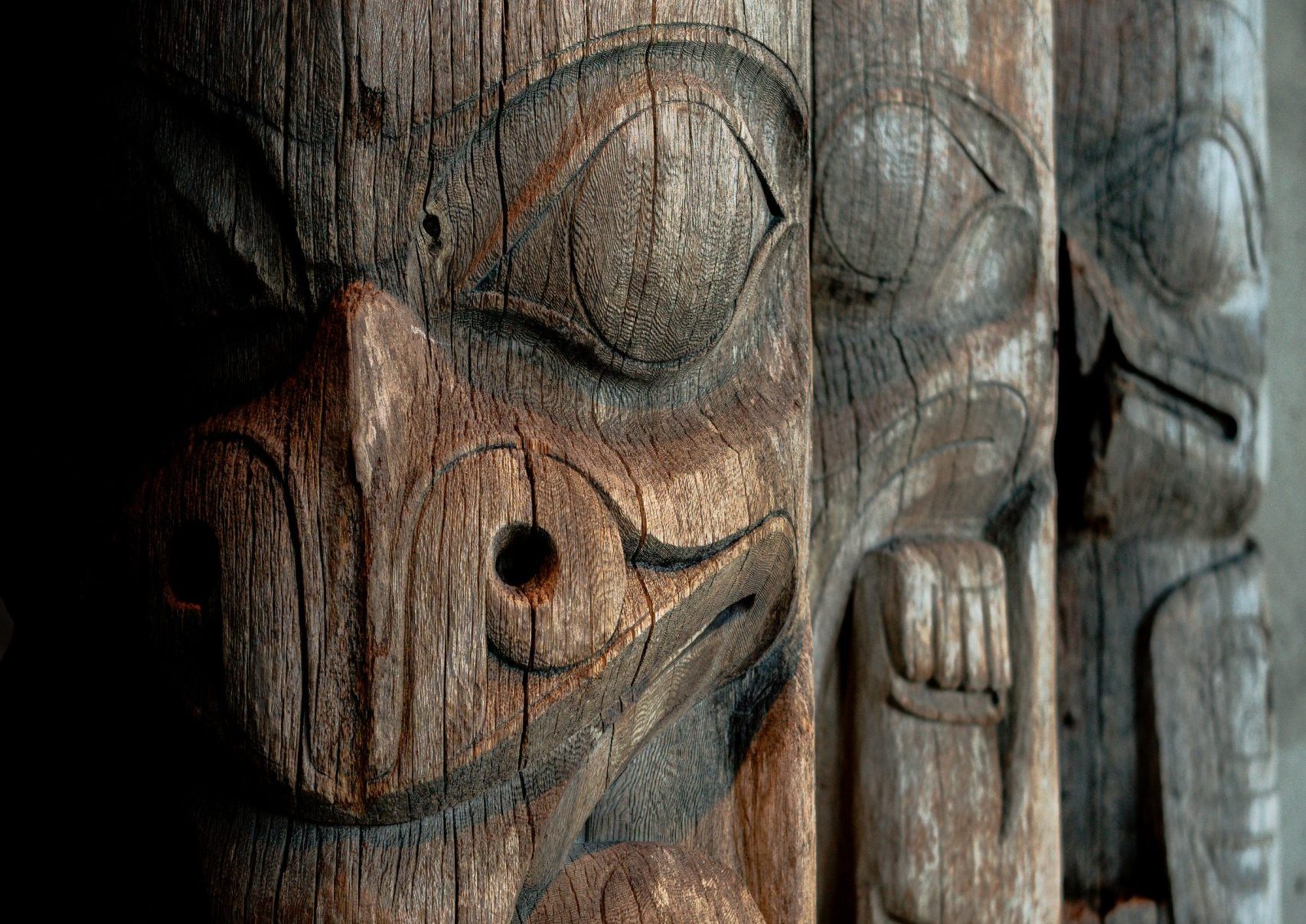The photograph showcases three intricately carved wooden totems, exuding an Alaskan totem pole style, all sharing a common textured smoothness without any chipping. The totem in the foreground, sharply in focus, is predominantly brown with the most vibrant reddish tones, suggesting it’s the newest. It features large, vivid eyes encircled by red, yellow, and blue stripes, resembling bird eyes. The nose is detailed with nostrils, shaped like an animal snout with a horn at the tip. Below, a meticulously carved mouth completes its face.

The second totem, partially obscured, is grayish. Although blurry, it reveals a design akin to the first but with slight variations in the mouth's depiction. Only one prominent eye and a part of the mouth are discernible, with a semblance of a large paw adding to its character.

The third totem, the lightest in color, presents itself from behind the others. Though it’s less visible, its distinguished features include a pronounced beak and a wing beneath it, enhancing the bird-like motif. This intricate tableau captures the beauty and craftsmanship of each totem's unique yet harmonizing elements.